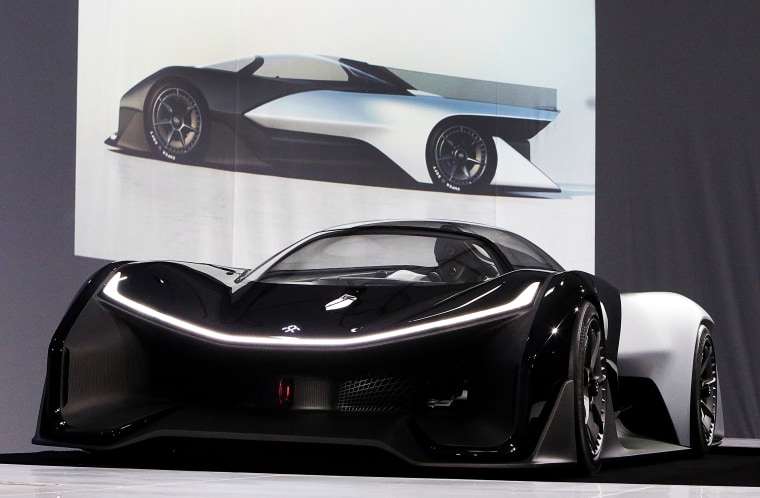This image features a sleek, black and white sports car, captured from a slightly angled perspective with the front of the car facing directly towards the viewer. The back tire is visible in the lower right corner of the image, showcasing the car's dynamic profile. The front end of the car is painted black, seamlessly blending into the polished white rear. Positioned in a showroom setting, the background features a gray curtain adorned with a sign depicting a side profile of the same car, adding to the futuristic and sophisticated ambiance of the scene. The car's immaculate finish and modern design elements highlight its innovative aesthetic.